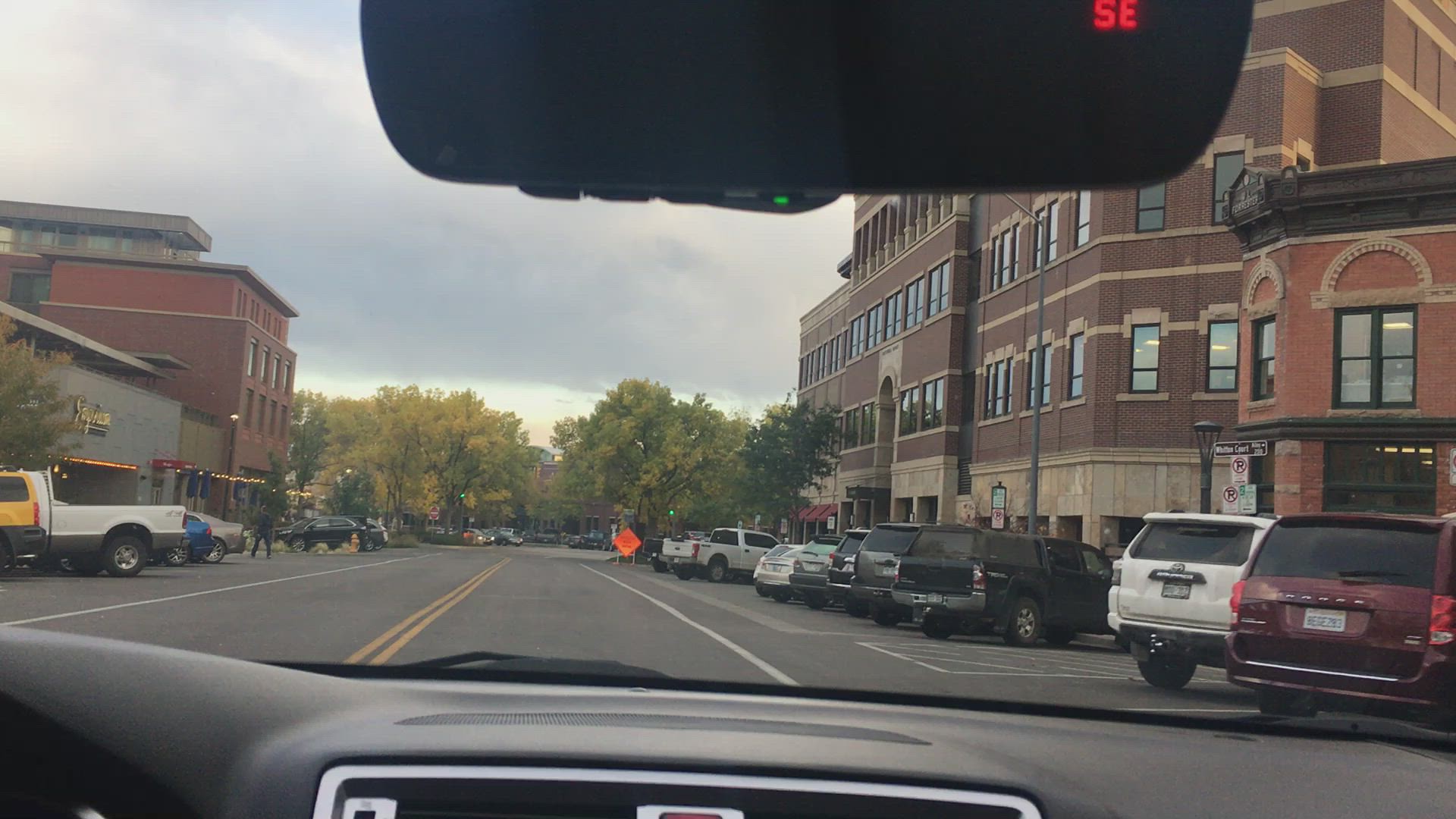The image captures a view from inside a car looking through the front window, where the black rearview mirror with red "SE" letters and a black dashboard with silver linings are visible. Ahead lies a dark grey road marked with double yellow lines down the center and white lines along the edges. On either side of the road, about a dozen large SUVs—colored red, black, white, and grey—are parked. Dominating the sides of the street are tall brown buildings with numerous windows, each featuring black linings, and an additional grey building on the left. In the distance, green trees line the horizon, while a bright, orange square sign turned on its side is affixed to posts on the roadside, although its message remains unclear.